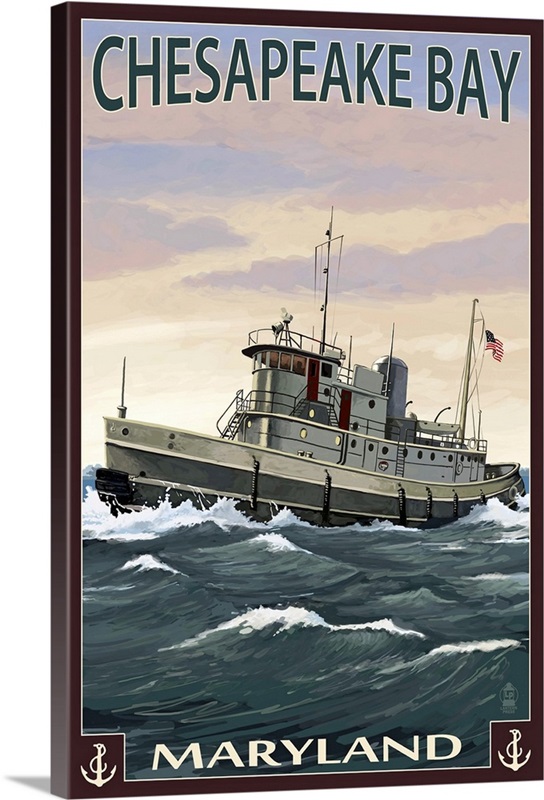This image depicts a vintage-style canvas panel print that could potentially be purchased as a souvenir in a gift shop for Chesapeake Bay, Maryland. The artwork features a deep burgundy trim and the title "Chesapeake Bay" at the top in a thick, dark green font. The background showcases a dramatic sky filled with shades of purple, pink, blue, and tan, suggesting a setting or rising sun behind pastel clouds. Below the sky, a large metal naval ship dominates the center, characterized by its art deco design with rounded, aerodynamic features, and an American flag flying proudly at its rear. The ship navigates through choppy, dark greenish-black waters, with the crests of waves vividly portrayed. At the bottom of the artwork, the word "Maryland" is boldly displayed in white font, flanked by naval anchors on either side, completing the composition. This detailed and evocative poster captures the essence of Chesapeake Bay with a blend of historical reverence and artistic flair.